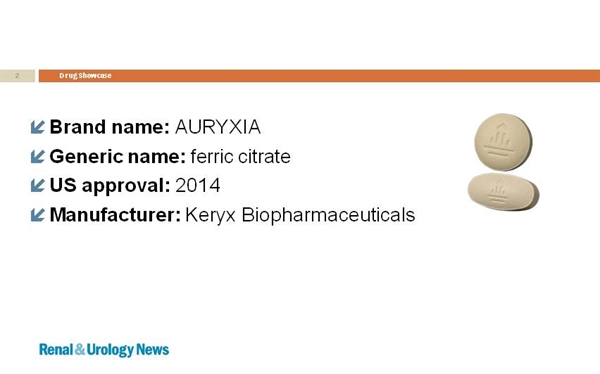Description: The image is a cropped screenshot of a website showcasing pharmaceutical drugs. 

At the top left, there is a warm gray rectangle containing the number "2". To its right, a small section reveals a white background, followed by an orange bar that extends to the right edge of the image. Within the orange bar, on the left side, the words "Drug Showcase" are displayed in white letters. 

The rest of the image has a white background and is divided into two columns. The left column features rows of text, each prefaced by a blue arrow pointing southwest. 

- The first row reads "Brand Name: Rexcauryxia" in bold letters.
- The second row states "Generic Name: aspheric citrate" with "Generic Name" in bold.
- The third row displays "U.S. Approval: 2014."
- The fourth row lists the "Manufacturer: Caryx Biopharmaceuticals."

The right column contains an image preview of the pills. There are two pills:
- The top pill is round with an imprint that is difficult to identify.
- The bottom pill is oval and thicker, with a similar, indistinguishable imprint.

At the bottom left of the image, "Renal and Urology News" is written in blue text.